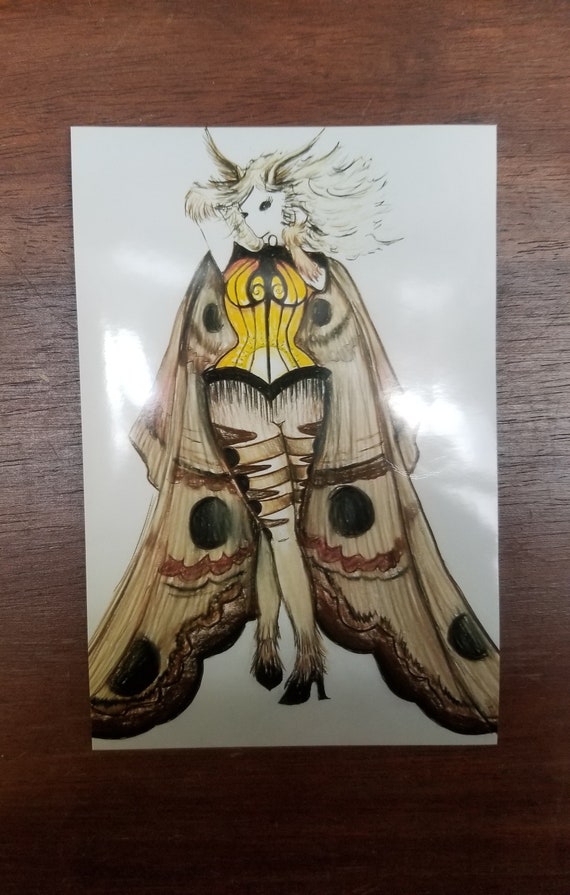In this photograph, a vivid drawing is displayed on a glossy white piece of paper, placed against a brown wooden surface, likely a floor or desk with a visible horizontal grain pattern. The drawing portrays a curvy, pretty human-moth hybrid with long, white-blonde hair and striking black eyes, but no nose or mouth. She dons a yellow top paired with black heels or possibly moth-like feelers and has distinctive hairiness at the bottom of her legs. Her expansive wings, adorned with black circular designs, extend broadly from her shoulders to the ground, resembling a cape in yellow-tan hues. The detailed rendering of the character, with its intricate wing pattern and glossy finish, highlights the artist's skillful technique.